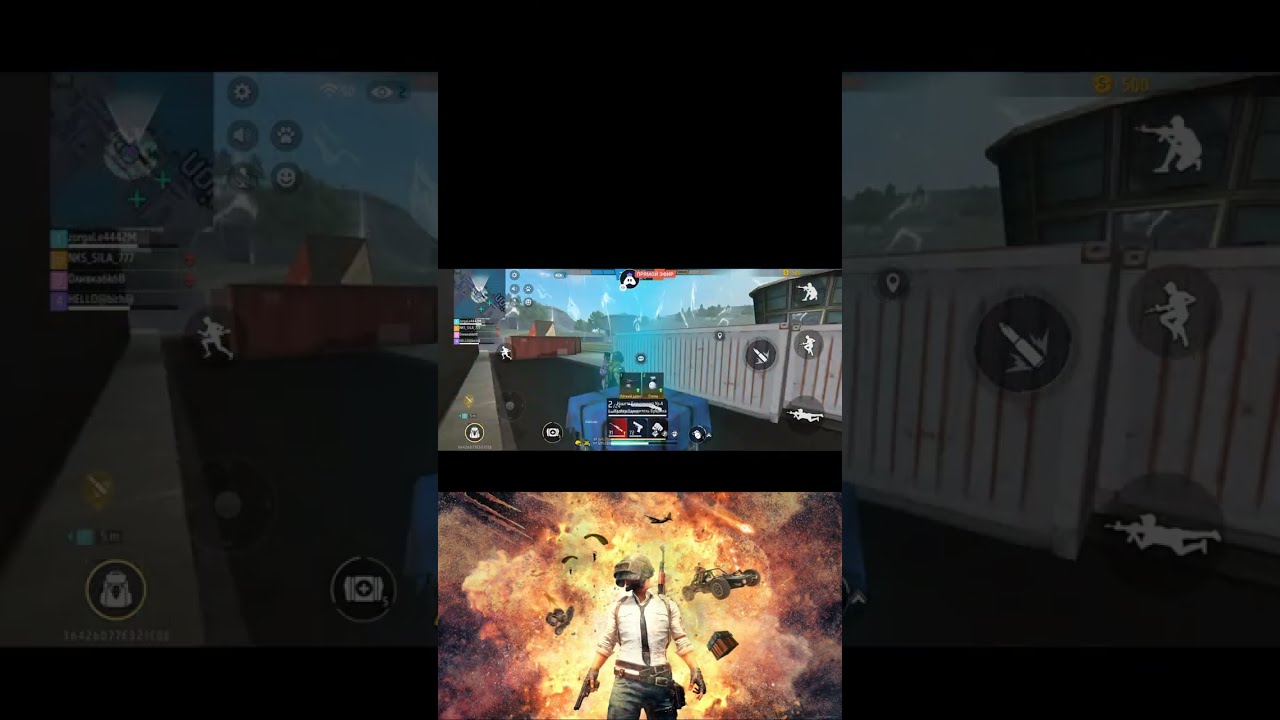The image, horizontally rectangular with grayed-out areas on the right and left sides, features three small rectangular sections in the center, presented vertically. The topmost section is dark and featureless, offering no distinguishable details. Below it, the middle section appears to depict a setting with boxcars and possibly an automobile, suggesting a storage or industrial area, with a hint of a white fence in the background. The bottom section is the most detailed, showcasing a dramatic scene of a man, presumably a superhero, standing amidst an explosion with flames in vivid red, orange, and yellow hues. He is dressed in a white collared shirt, a thin black tie, and dark pants. Notably, he has two brown leather belts with large silver buckles around his waist, and a pouch hangs from one. The man, also wearing a welder's mask and fingerless gloves, holds a weapon, likely a gun, in one hand. Surrounding him are various pieces of flying debris, including a car and a box, accentuating the chaotic explosion behind him.